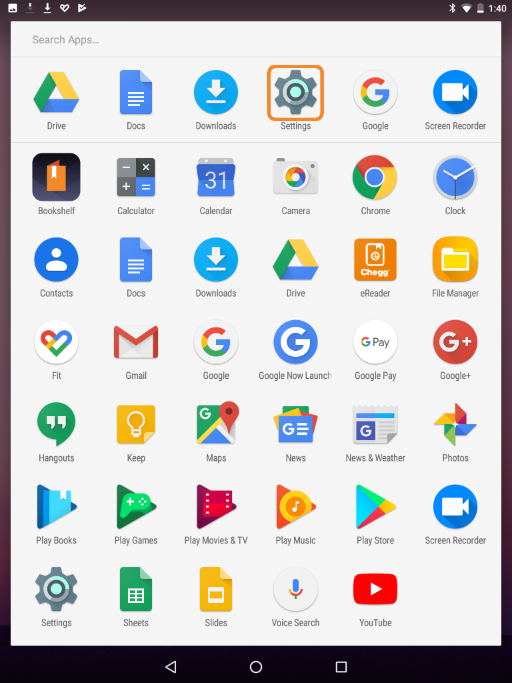The image depicts a smartphone screen with a plethora of details. Enclosed within a square frame, the uppermost section of the screen features a black border housing five icons. To the right of this area, additional icons are displayed, including indicators for Bluetooth, Wi-Fi signal, and battery status, which notably shows approximately one-eighth of battery life remaining. The time displayed on the phone is 1:40.

The main portion of the screen is occupied by a grid of app icons arranged in six rows across and seven columns down, filling the entire screen save for the lower right corner, which is noticeably empty. At the very bottom of the screen, there are three essential navigation icons in white: an arrow for going back a page, a circle likely representing the home screen, and a square icon.

Specifically, the top left corner features the Google Drive app, while the settings app is located towards the lower part of the screen. The last app icon on display is YouTube. The organized layout and specific details provide a comprehensive snapshot of this smartphone's interface.